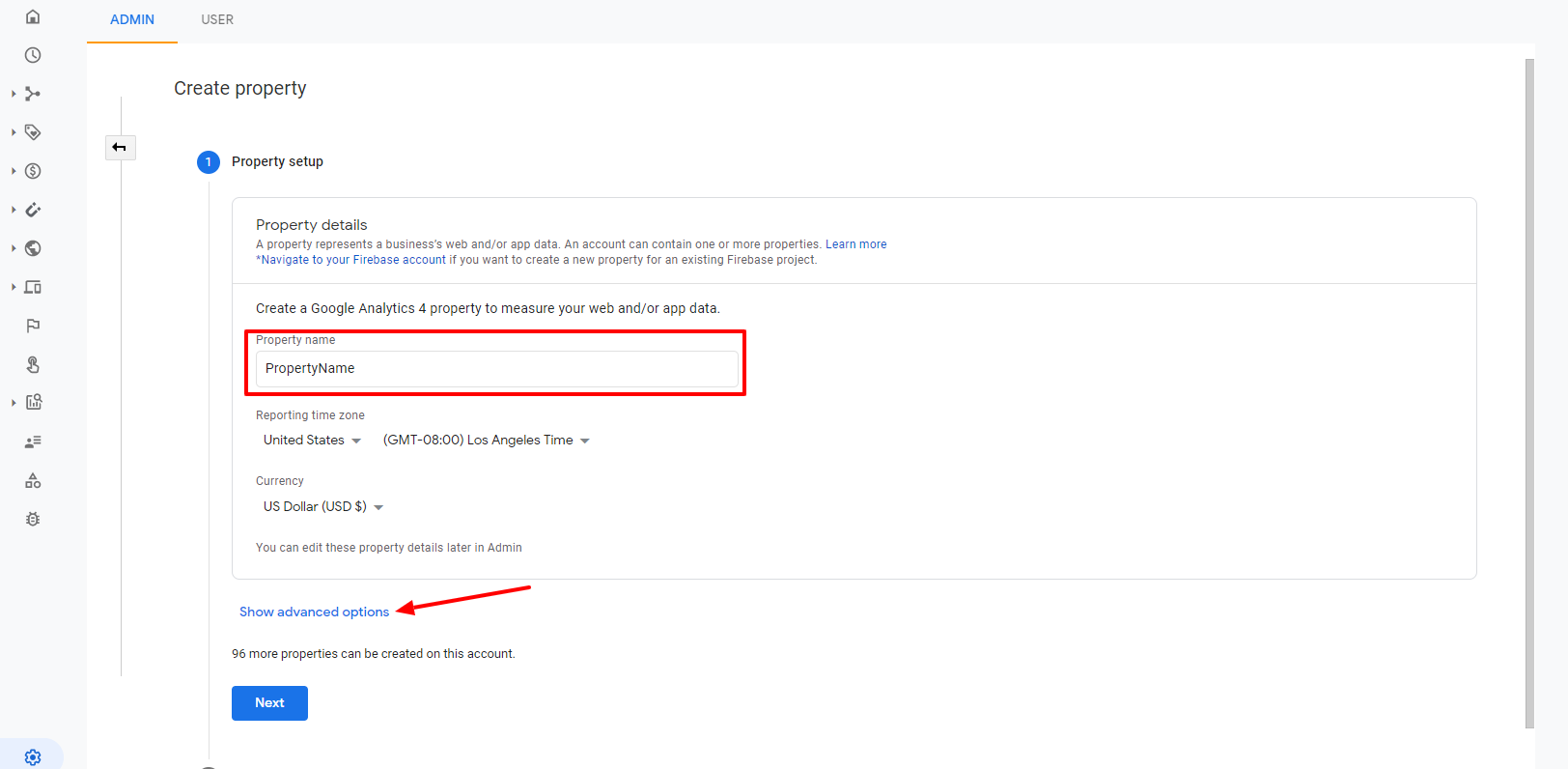Screenshot of an interface for creating a property listing:

On the left-hand sidebar, a series of icons are vertically aligned against a gray background. These icons include:

1. An outline of a house
2. A clock
3. A tag symbol, often associated with a sale
4. A circle containing a dollar sign
5. A magnet
6. A globe representing the world
7. A smartphone and laptop
8. A flag
9. A book
10. A finger pressing a button
11. A bar graph with a magnifying glass over it
12. A person examining a document
13. Shapes including a triangle, square, and circle
14. An image of a bug
15. At the bottom left, there is a blue gear icon

At the top of the sidebar, the word "Admin" is displayed in white and underlined in orange, with "User" written in gray beneath it. 

In the main section, a white box with black text reads "Create Property." Below it, there is a blue circle with a white number one inside next to the heading "Property Setup." Under this heading, sub-categories include:
- Property Details
- Property Representation

There is also a section inviting the user to "Create a Google Analysis for property to measure your web and/or map data."

A red rectangle labeled "Property Name" features a text box where "Property Name" has been entered. An arrow nearby points to a link in blue that reads "Show advanced properties."